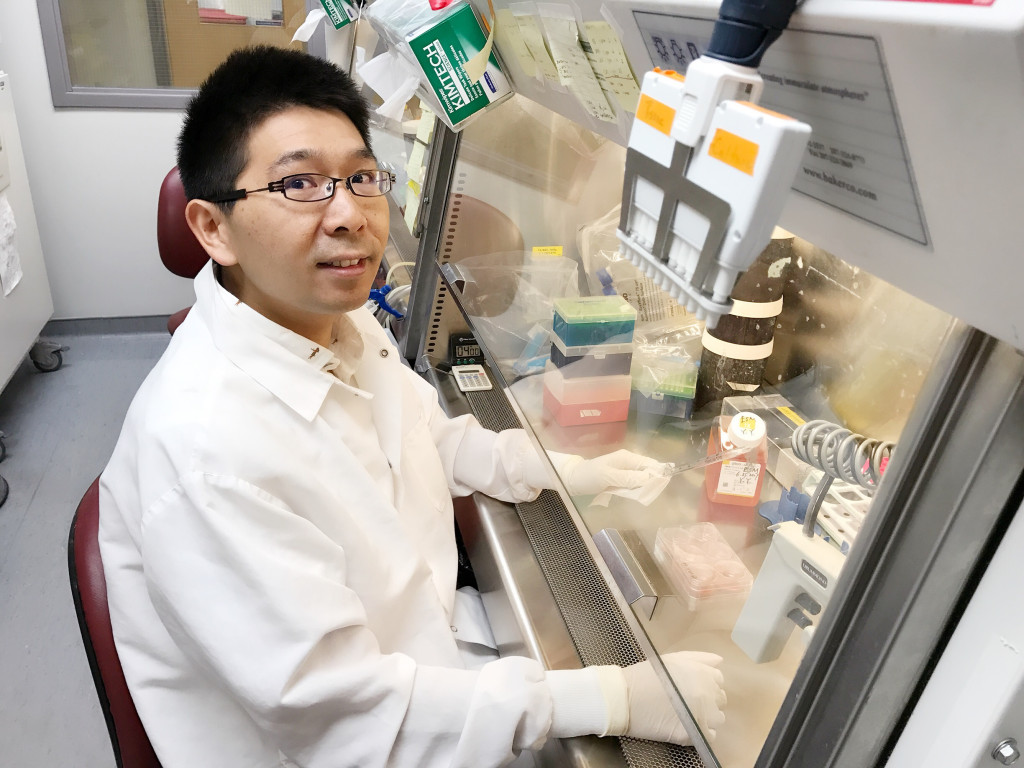The photograph captures a detailed scene inside a sterile science laboratory. A young man, possibly a scientist or technician, with short black hair and black-rimmed glasses, is seated in a red leather rolling chair. He is wearing a white lab coat and white gloves. The man is engaging with a sophisticated piece of lab equipment—a metallic and glass cabinet with a clear glass partition that is lowered to accommodate his hands. This setup ensures a sterile environment for his experiment. 

His hands are inside the cabinet, which contains various colored containers—black, blue, clear white, and red—and several intricate instruments, including what appears to be a silver scalpel and a red sharps container. Behind him, the lab is adorned with a variety of technical equipment and containers, contributing to an overall sense of a meticulously organized workspace. The background features sterile white walls, a grey-trimmed large window, and a gray floor, reinforcing the clinical atmosphere of the lab. The man is looking up at the camera and smiling slightly, as he continues his precise lab work.